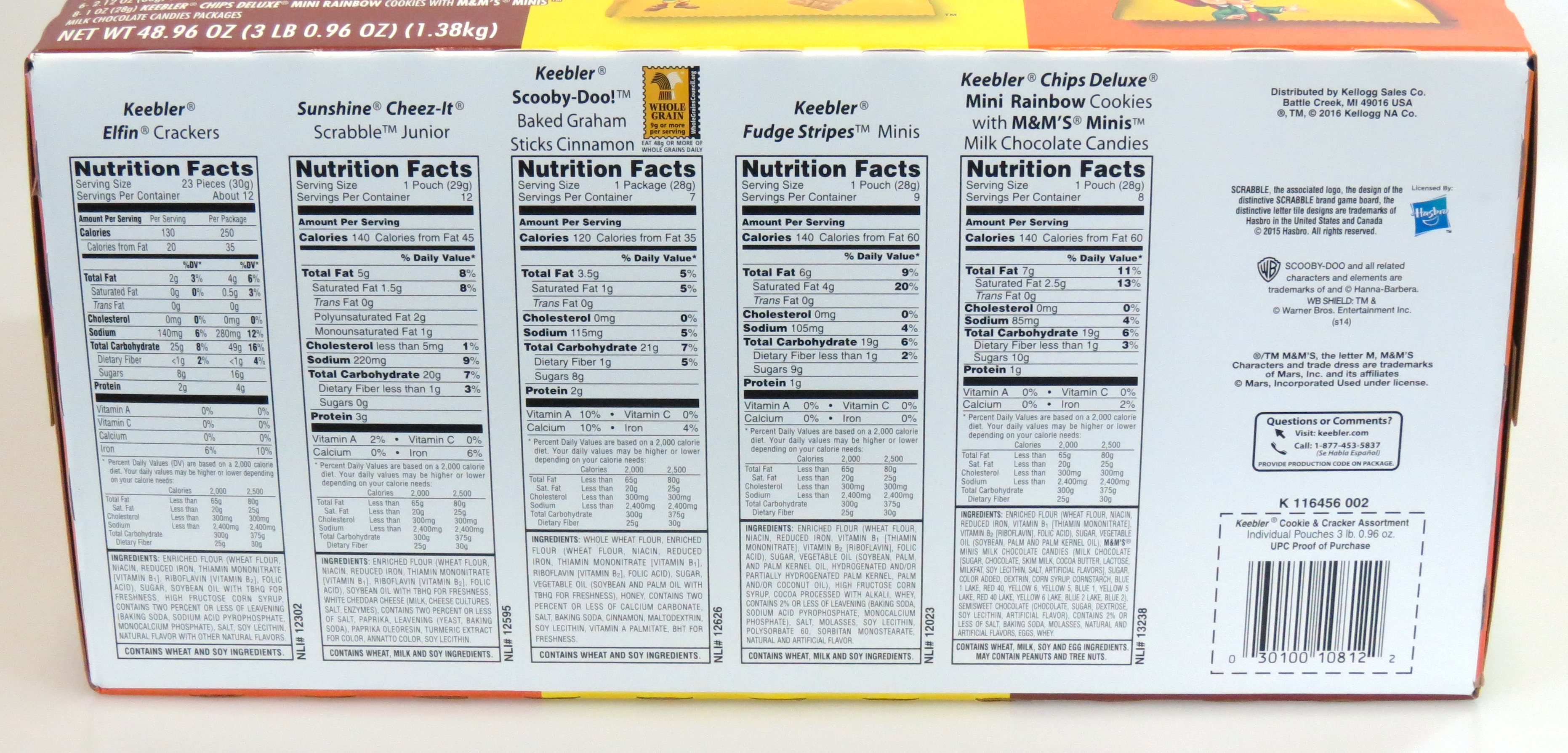This detailed photo captures the bottom side of a rectangular cardboard box containing a variety pack of snacks. The box is positioned on its right side, displaying a vertical arrangement of nutrition facts labels for the included snacks. Visible at the top of the image is a portion of the left side of the box, featuring a maroon rectangle that lists the weights of the individual snack packages.

On the left side of the photo, two partial images of snack packages are visible. The first, from the left, has a yellow background and shows the bottom segment of the package, while the second, on the far right, has an orange background with a small yellow section of the package in view.

The back of the box prominently features the names and nutritional information of the snacks in vertical rectangles. They are listed as follows:
1. **Keebler Elfin Crackers** - with the nutritional facts provided below.
2. **Sunshine Cheez-Its Scrabble Jr.** - followed by its nutritional panel.
3. **Keebler Scooby-Doo Baked Graham Sticks Crackers** - displaying an icon for whole grains beside it, with the nutritional facts beneath.
4. **Keebler Fudge Stripes Minis** - with its nutrition information.
5. **Keebler Chips Deluxe Mini Rainbow Cookies with M&Ms Minis, Milk Chocolate Candies** - with the corresponding nutritional panel below.

The right side of the box contains a densely written area, including a section labeled "Questions or Concerns," accompanied by a telephone number and website address. Adjacent to this, within a dashed outline, is a prominent barcode.

This image provides a comprehensive view of the product information for the various snacks inside the mixed box, ensuring consumers have access to detailed nutritional data at a glance.